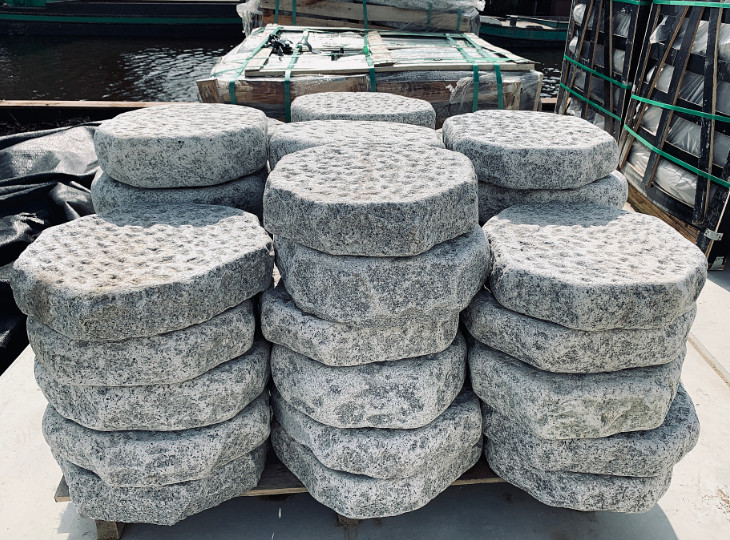The image captures a storage yard by the water, presumably a shipment facility, in broad daylight. The central focus is a collection of decorative garden stones that have been meticulously stacked on wooden pallets. These stones are hexagonal in shape, crafted to mimic a weathered appearance, likely made from brick or cement. The stacks vary in height: the left and right stacks each have five stones, the middle stack has six, and there seem to be additional stacks behind these initial three, totaling approximately 40 stones. Each stone is textured with tiny divots, likely intended to provide grip and prevent slipping when used as stepping stones in a garden pathway. Surrounding the main stacks, there are other items wrapped in plastic or secured in wooden crates, indicating readiness for shipment. The backdrop reveals a waterway, possibly a canal, suggesting close proximity to a loading or unloading area.